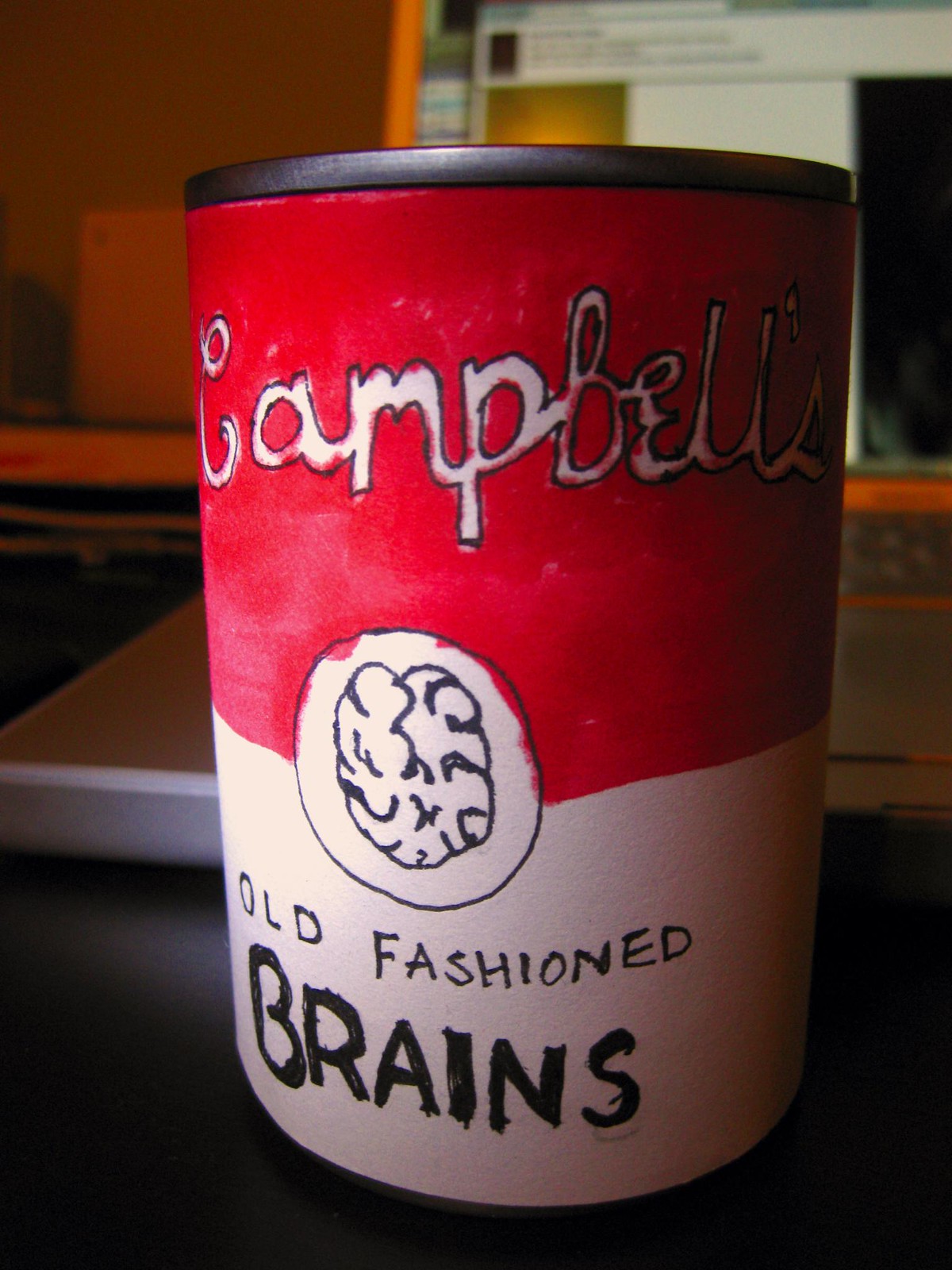This close-up image features a soup can with a custom-made label designed to mimic the iconic Campbell's soup can. The can itself is a dark silver color, providing a stark contrast to the vibrant label. The label is split horizontally with the upper half painted red and the lower half white. At the top, "Campbell's" is written in elegant, cursive white lettering outlined in black, capturing the classic look of the original branding. Below, in bold black lettering, the label reads "Old Fashioned Brains," adding a whimsical touch. Centered on the label is a white circle straddling both the red and white sections, inside of which is a detailed, hand-drawn illustration of a brain. The can is placed on a sleek black tabletop, further accentuating the creative and playful detail of the label.